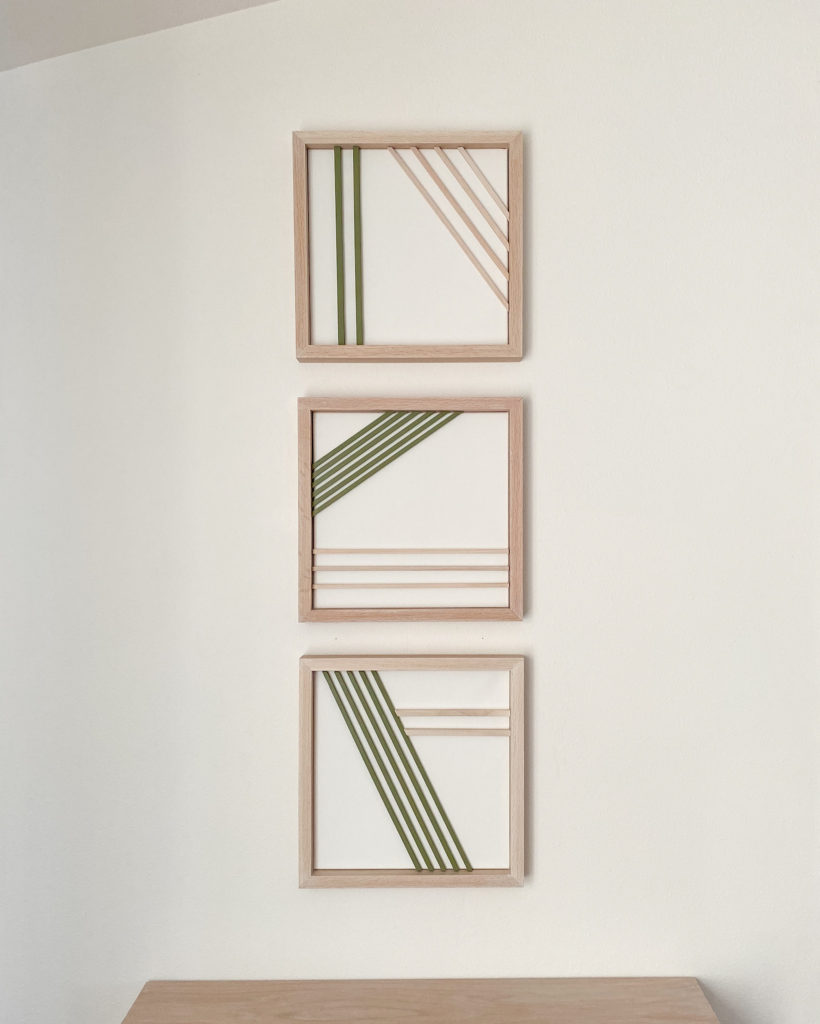In this contemporary indoor setting, three pieces of framed abstract wall art are vertically aligned on a pristine white wall. Each piece is enclosed in a bleached wood frame, mirroring the finish of the wooden table below. The artwork is characterized by its minimalist design, featuring a series of stripes in black, beige, and gray. 

The top frame presents two black vertical stripes on the left, juxtaposed with a triangular formation of beige stripes in the corner. The middle piece, positioned directly beneath, displays black stripes arranged diagonally from the middle left to the top right corner and intersecting beige stripes from the bottom left. Finally, the bottom frame showcases a large central black stripe extending vertically, accompanied by two smaller beige diagonal lines on either side. The beige hues in the artwork seamlessly match the color of the frames, creating a cohesive and modern aesthetic. The entire setup exudes a sense of simplicity and elegance, enhanced by the contrast of the natural wood against the crisp white background.